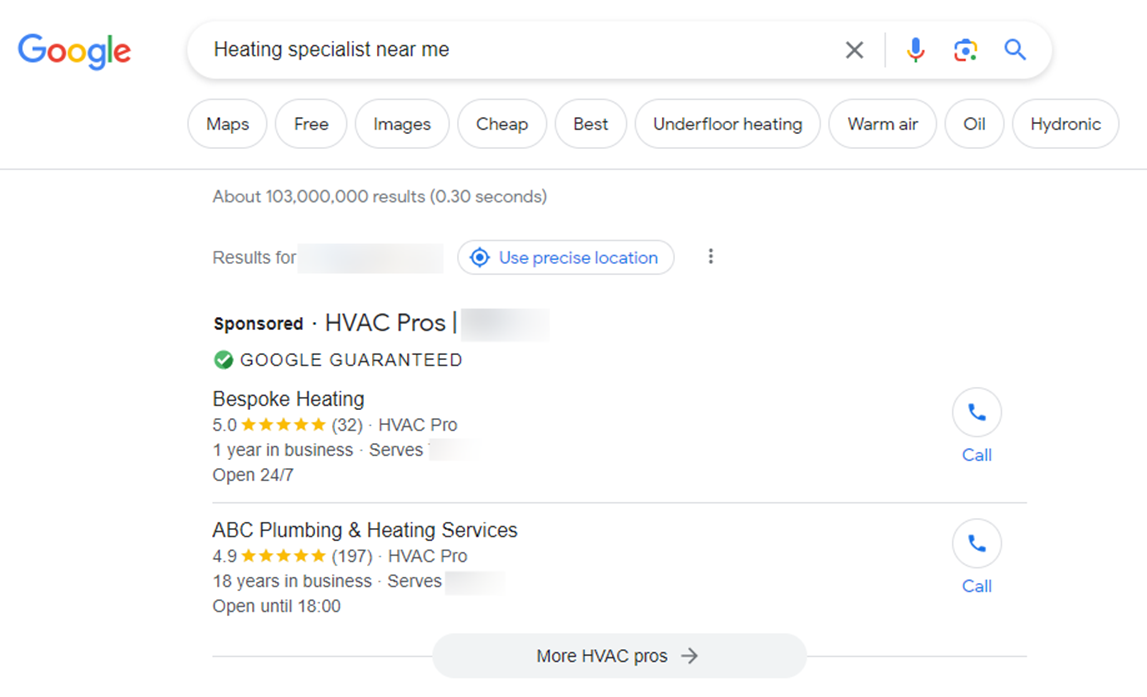The image shows a Google search results page with the query "heating specialist near me." In the upper left corner, the iconic Google logo is displayed in its usual colors: blue, red, yellow, and green. To the right of the logo, the search bar stretching across the page contains the typed query "heating specialist near me." Next to the search bar on the right, there is an 'X' icon for clearing the search, followed by a vertical line and a multicolored microphone icon similar to the Google logo, which is used for voice search. To the right of this, a camera icon with rainbow colors (indicating Google Lens) is present, and finally, a magnifying glass icon for initiating the search.

Below the search bar, a navigation menu includes options such as "Maps," "Free," "Images," "Cheap," "Best," "Underfloor Heating," "Warm Air," "Oil," and "Hydronic." Beneath this menu, a line separates the navigation from the search results. The results section starts with a note indicating approximately 103 million results found in 0.30 seconds.

The first section of results is blurred, but an option to "Use precise location" is visible in an oval box on the right, alongside its corresponding icon and a three-dot menu for additional options. The word "Sponsored" appears next, indicating paid advertisements or listings.

The first sponsored result is for "HVAC Pros," featuring a brief description of bespoke heating services and ratings, accompanied by a call icon on the right. Below this, there is another listing for "ABC Plumbing and Heating Services," which also includes rating information and a call icon. At the bottom of the listed results, a "More HVAC Pros" button with a right arrow invites users to view additional service providers.